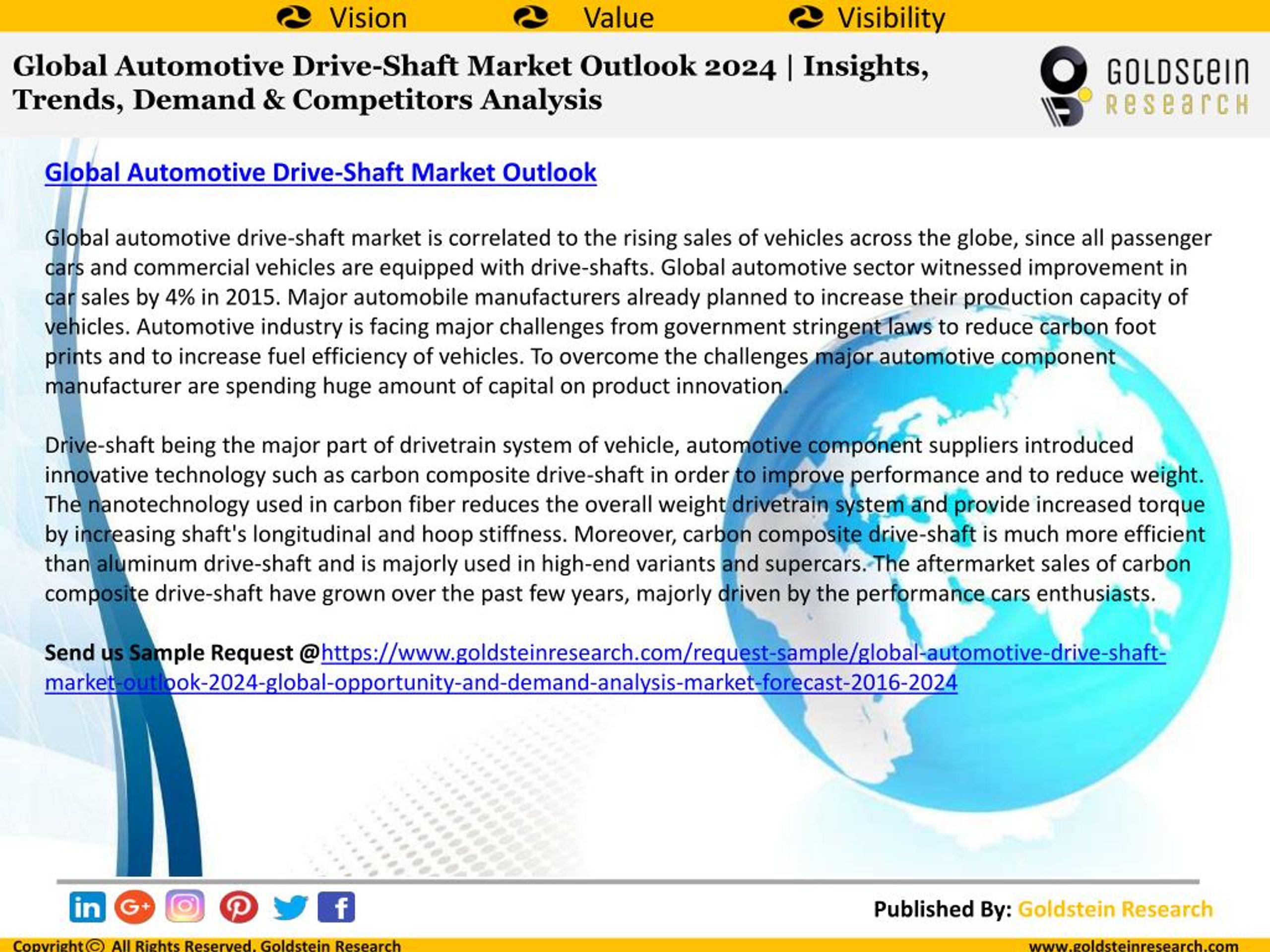**Detailed Image Caption:**

The image originates from GoldsteinResearch.com, focusing on the "Global Automotive Driveshaft Market Outlook for 2024." At the top of the image, the text "Vision, Value, Visibility" is prominently displayed. To the right, the Goldstein Research logo features the words "Goldstein" in black and "Research" in a yellowish-green color, situated below an emblem. This emblem consists of a black circle, a yellow circle, and a left-facing magnet icon.

The main heading reads "Global Automotive Driveshaft Market Outlook 2024," followed by a subheading that includes "Insights, Trends, Demand, and Competitors Analysis." The caption text elaborates on the role of the global automotive driveshaft market, emphasizing its correlation with rising vehicle sales worldwide. It details how all passenger cars and commercial vehicles are equipped with driveshafts and notes a 4% improvement in car sales in 2015. This growth has prompted major automobile manufacturers to increase their production capacity. 

The text also highlights the industry's challenges due to stringent government regulations aiming to reduce carbon footprints and increase fuel efficiency. To address these challenges, automotive component manufacturers are investing significantly in production innovation. The second paragraph discusses the importance of driveshafts as a crucial component of a vehicle's drivetrain system. It highlights innovations such as carbon composite driveshafts which improve performance and reduce weight. The use of nanotechnology in carbon fiber driveshafts decreases the overall weight of the drivetrain system and improves torque and shaft stiffness. 

The superior efficiency of carbon composite driveshafts over aluminum ones, particularly in high-end supercar variants, is noted. Additionally, the aftermarket sales of carbon composite driveshafts have surged due to demand from car enthusiasts. The image includes a prompt to request a sample, directing viewers to a URL for the sample request.

The background of the image is white, featuring an illustration of the Earth, showcasing continents from Africa to Asia and Europe, with white land masses and blue oceans. Social media icons for Twitter, Pinterest, and Facebook are visible at the bottom, and the text "Published by Goldstein Research" is located in the lower right corner.